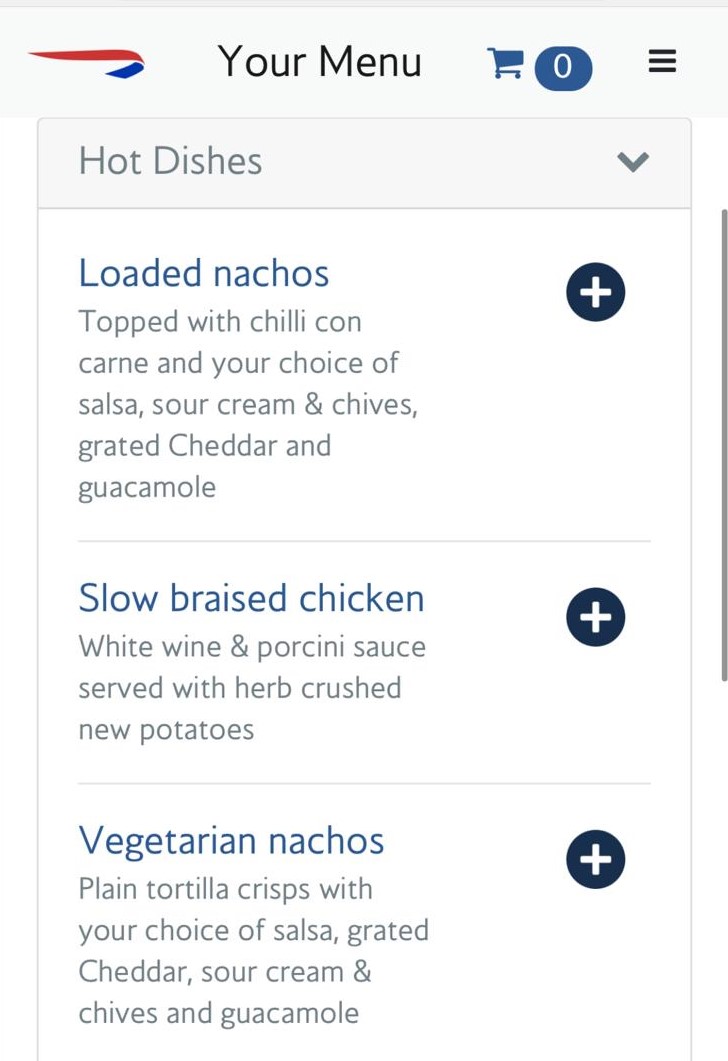This image, likely viewed on a mobile device due to its vertical orientation, features a website layout. At the top left corner, there is a red and blue logo resembling a streaming flag, signifying the website's branding. Adjacent to the logo, the title "Your Menu" is prominently displayed. 

To the right of the title, a blue shopping cart icon indicates the number zero, suggesting an empty cart. Further right, three stacked lines (a common menu icon) imply a drop-down menu, although it's currently not expanded. 

Beneath these elements, a gray label reads "Hot Dishes" accompanied by a down arrow, hinting at a dropdown selection. Below this, three menu options are visible, with each dish name highlighted in blue and accompanied by a plus symbol for adding them to the cart. 

The first option, "Loaded Nachos," is topped with chili con carne and offers a selection of salsa, sour cream and chives, grated cheddar, and guacamole. 

The second dish, "Slow Braised Chicken," comes with a white wine and porcini sauce and is served with herb-crushed new potatoes.

The final option is "Vegetarian Nachos," which are plain tortilla crisps available with salsa, grated cheddar, sour cream and chives, and guacamole. A scroll bar on the right suggests additional options are available beyond the current view.